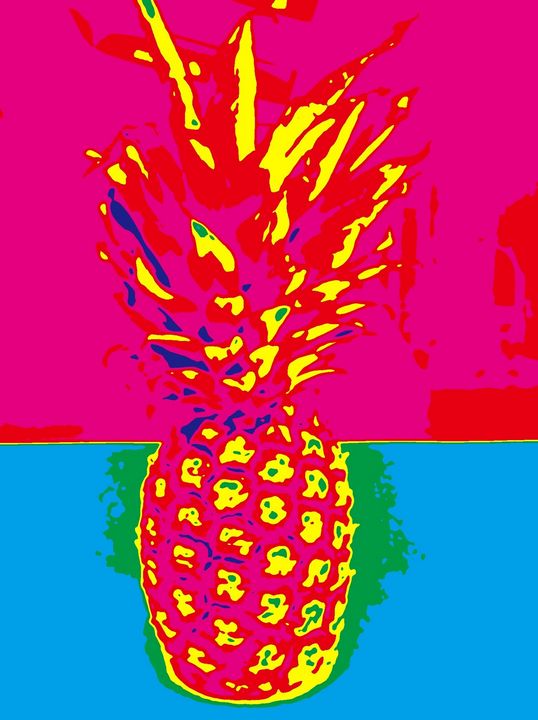This vibrant, neon-colored illustration of a pineapple features a bold, graphic, almost cartoony aesthetic. The image is dramatically split vertically in terms of color: the top half is dominated by hot pink and red hues, while the bottom half showcases bright blue with splotches of green. The pineapple itself is highly saturated with intense colors, including shades of hot pink, red, bright yellow highlights, and touches of green. The shadows are depicted in dark blue, adding depth without sacrificing the illustration’s simplicity. The overall artistic style is far from realistic, embracing saturated, simple colors, and minimal, though clear, details. The bright, energetic color scheme and sharp tonal division of the background further amplify the dynamic, heavily edited feel of the artwork.